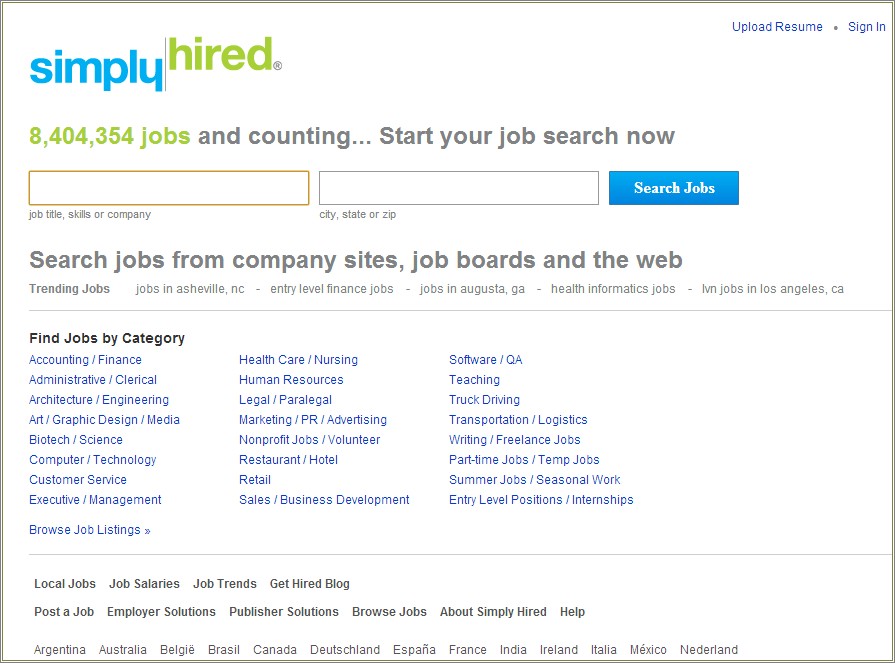A screenshot of the SimplyHired homepage reveals a minimalistic design reminiscent of Craigslist, highlighting simplicity and ease of use. Prominently displayed is a bold statement proclaiming "8,404,000 jobs and counting," encouraging users to "Start your job search now." The layout is straightforward, featuring a search bar where users can input a job title, skills, or company, alongside a city, state, or zip code to refine their search. A conspicuous blue "Search Jobs" button invites users to dive into the job hunt. 

In the top right corner, options to upload a resume or sign in are conveniently placed for easy access. Below the search bar, a categorized list of job sectors is presented, ranging from accounting, administration, and architecture to customer service, healthcare, legal, marketing, and more. This extensive list showcases various employment structures, including freelance, part-time, full-time, entry-level, and summer jobs, catering to a wide array of job seekers. 

Near the bottom of the page, additional links provide insights into salaries and job trends, alongside access to a blog aptly named "The Get Hired Blog," offering tips and advice for job seekers.